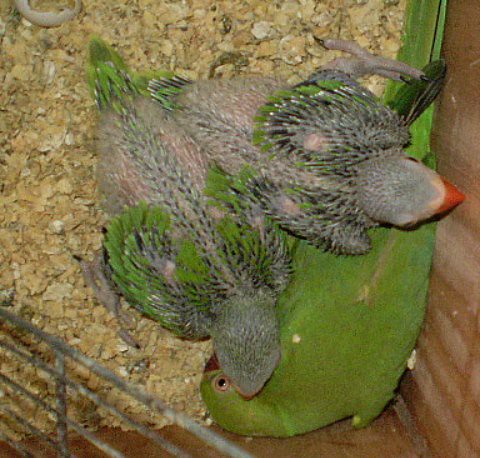The photograph captures a detailed scene inside a birdcage viewed from above. The image prominently features an adult green parrot with an orange beak, lying in the lower corner, surrounded by wood shavings, hay, and birdseed hulls scattered on the cage floor. Nestled on top of the adult bird are two tropical chicks, appearing mostly naked with patches of emerging green feathers on their wings and tails, and grayish skin. The chicks have short orange beaks, although one chick's beak is not visible. The lower left-hand corner of the image shows the metal bars of the cage, while the right-hand side features a solid wood surface. There is a part of a cracked eggshell in the upper left-hand corner, adding to the intricate details of the cage's interior.